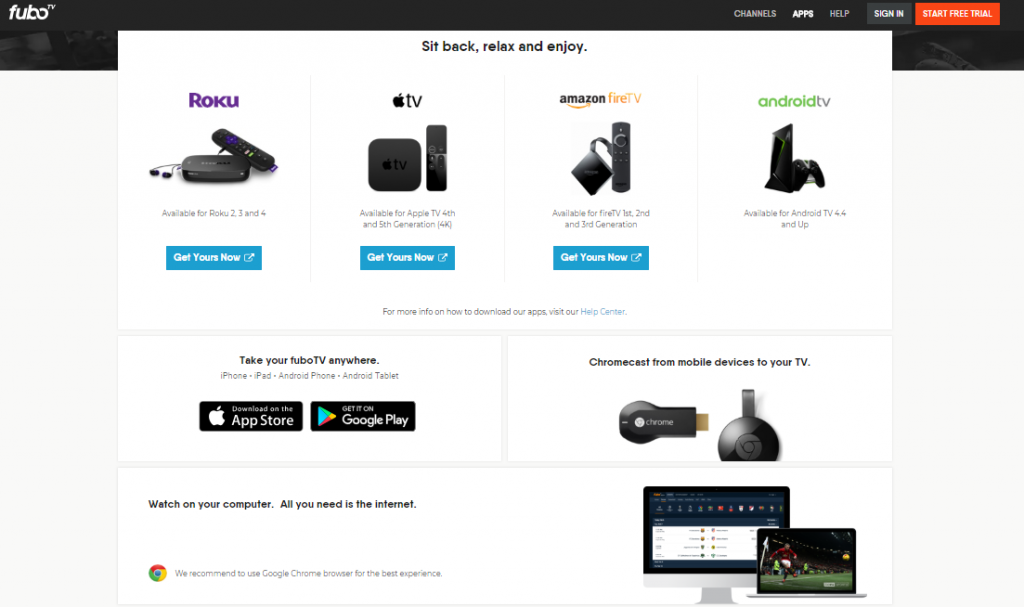The image features a sleek interface set against a black background. At the top left, "FUBO" is written in a flowing cursive font, accompanied by "TV" in smaller, adjacent white text, altogether reading "FUBO TV." 

On the left side of the screen, a menu lists the options: "Channels" in gray, "Apps" in white, "Help" in gray, and a prominent "Sign In" button in white, followed by an orange button with white text saying "Start Free Trial!" 

A pop-up window appears, with the message "Sit Back, Go Back, Sit and Enjoy!" rendered in black text. 

Below the pop-up, a lineup of streaming devices is showcased: a Roku player with the Roku logo in purple, an Apple TV with the iconic Apple logo in black, a Flare TV displaying the Amazon logo with "Flare TV" in orange, and an Android TV box marked by the green Android logo and gray "TV."

Additionally, the image advises, "For more information on how to download our apps, visit our Help Center." Beneath this text, there's a section promoting FUBO TV's compatibility with various devices: iPad, iPhone, Android phone, and Android tablet. Users are encouraged to download the app from the App Store or Google Play and are informed that they can Chromecast from mobile devices to their TV.

Images of Chromecasts, two generic MacBooks, and a suggestion to use Google Chrome for the best viewing experience on a computer are also included. 

Overall, the interface emphasizes the versatility and accessibility of FUBO TV across multiple platforms.